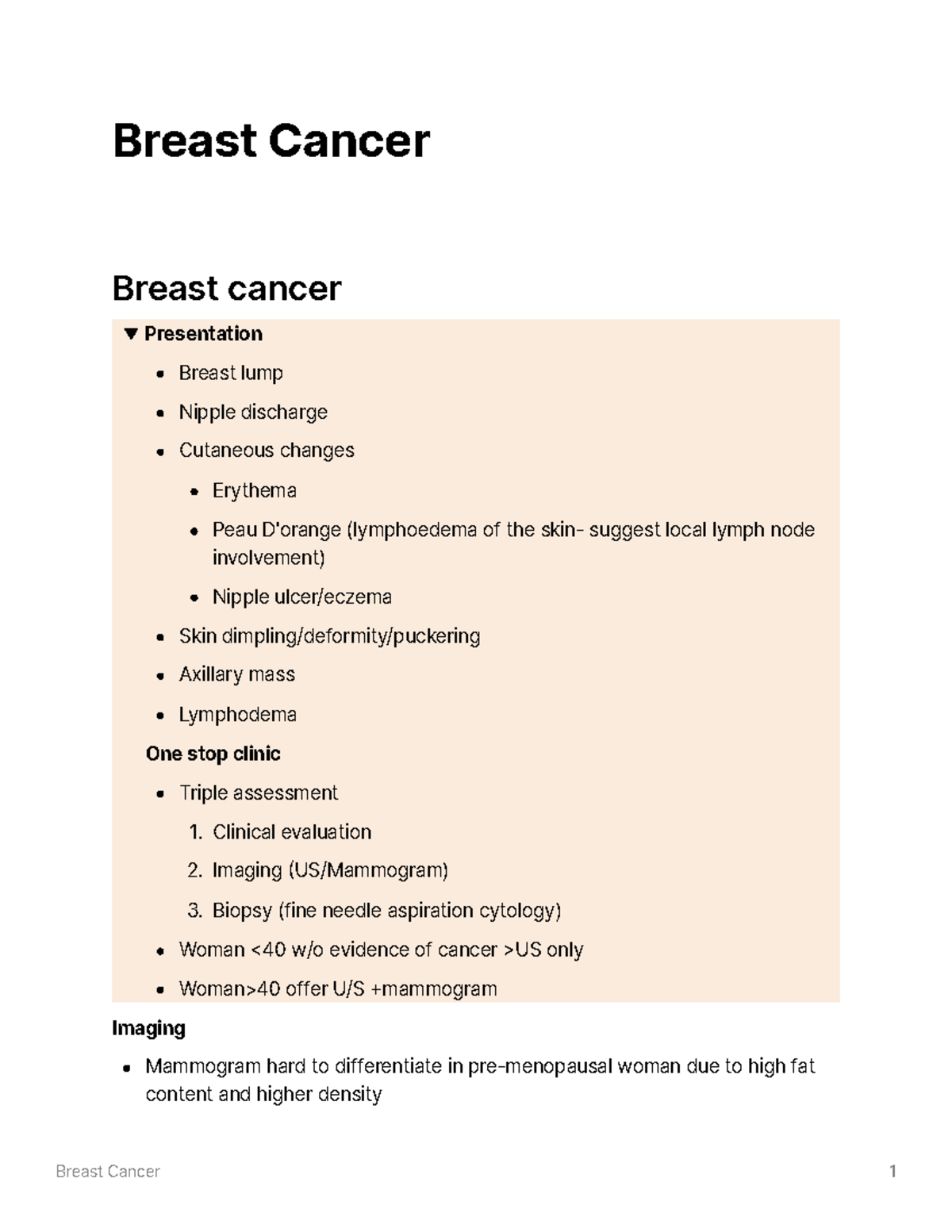**Detailed Caption:**

The image is a detailed screenshot presenting information on breast cancer, primarily featuring black text against a white background. The layout is vertically elongated but not very wide. At the top left corner, the title "Breast Cancer" is displayed prominently in large, bold, sans-serif letters. 

Below the title, after a significant blank space, “Breast Cancer” is repeated in smaller yet still bold font. This second instance of the title introduces a section outlined by a light pink box containing the following information in black text:

1. **Presentation (Subheading)**
   - Accompanied by a downward-pointing triangle. 
   - Bullet points:
     - Breast lump
     - Nipple discharge
     - Cutaneous changes
       - Sub-bullets:
         - Erythema
         - Peau d'orange lymphedema of the skin
         - Local lymph node involvement
       - Nipple ulcer / eczema
     - Skin dimpling, deformity, puckering
     - Axillary mass
     - Lymphedema

2. **One-Stop Clinic (Subheading)**
   - Bullet points:
     - Triple assessment
       - Sub-bullets labeled 1 to 3:
         1. Clinical evaluation
         2. Imaging (U.S./Mammogram)
         3. Biopsy (Fine Needle Aspiration Cytology)
     - Women < 40 without evidence of cancer (U.S. only)
     - Women > 40, offer U.S. + Mammogram

The pink box concludes here, giving way back to the white background.

3. **Imaging (Subheading)**
   - Bullet points:
     - Mammogram is hard to differentiate in premenopausal women due to high fat content and higher density.

At the very bottom of the image, there is another space followed by the last instances of text:
- On the bottom left, “Breast Cancer” appears again in a small, light gray font.
- On the bottom right, the number “1” is presented in the same small and light gray font.